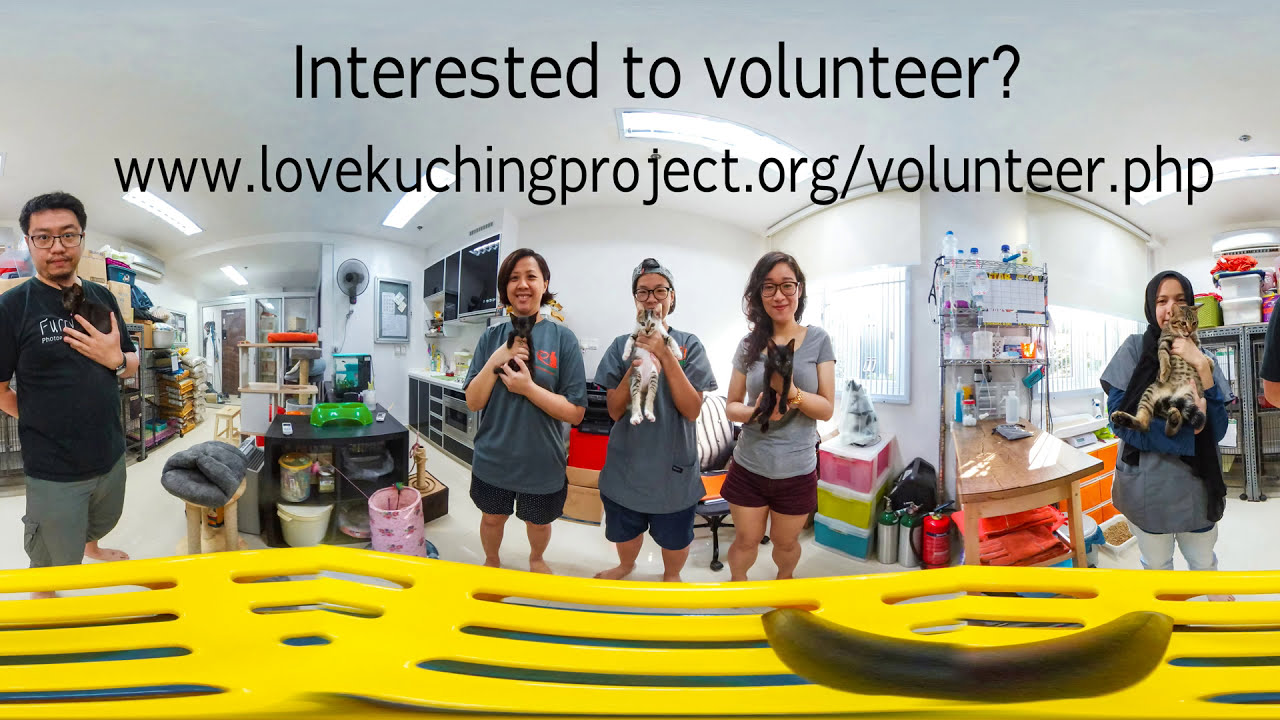In a 360-degree panoramic image, an Asian man in a short-sleeved black t-shirt with white writing and gray cargo shorts appears twice: his upper arm and elbow are on the right edge, while his full body, except for those parts, is on the left. He is barefoot and holding a black cat. Centrally, three Asian women, all wearing gray t-shirts and shorts, hold cats. Two wear glasses and one a cap. Their cats are a black cat, a black-and-white spotted cat, and another black cat, respectively. On the far-right side, an Asian woman in a hijab, gray smock, and tan pants holds a calico kitten. The white-walled background has various shelves and a glass door, suggesting a pet clinic or shop. A black table with grooming tools is on the left, and an examination table is on the right. A strip of yellow plastic with lattice work runs across the bottom, and in print it reads, "Interested to volunteer? www.lovekuchingproject.org or www.lovekoachingproject.org." The image concludes with a note from a webinar inviting questions and providing a contact number: 1-800-325-4242.